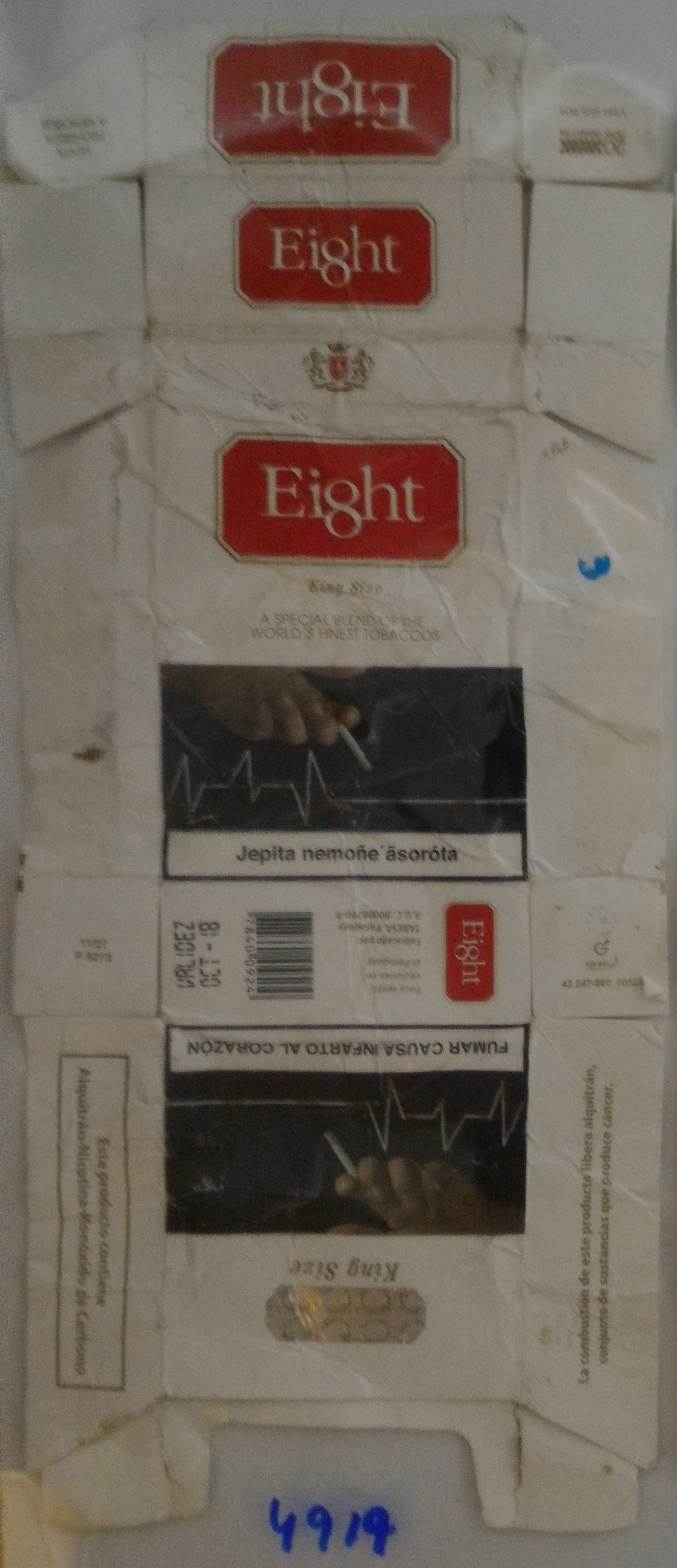This is a vertically cropped, blurry, and poor-quality photograph of what appears to be an unfolded and flattened cigarette package placed on a surface. The worn box is marked by various distinct design elements and colors, including white, red, black, and gold. Dominantly, it features a maroon-colored rectangle with the word "EIGHT" spelled out in white typeset. Below this, there's a photograph of a hand holding a cigarette with an electrocardiogram line underneath it, suggesting a health warning. Additional text is visible, though difficult to decipher, and one part indicates "king size" upside down. A bold blue marker inscription, "4919," is noticeably written at the very bottom, seemingly on a glass slide beneath the packaging. The labels and designs include a solid black area with white and gold elements, as well as segments with vertical stripes in red, white, gray, and gold colors.